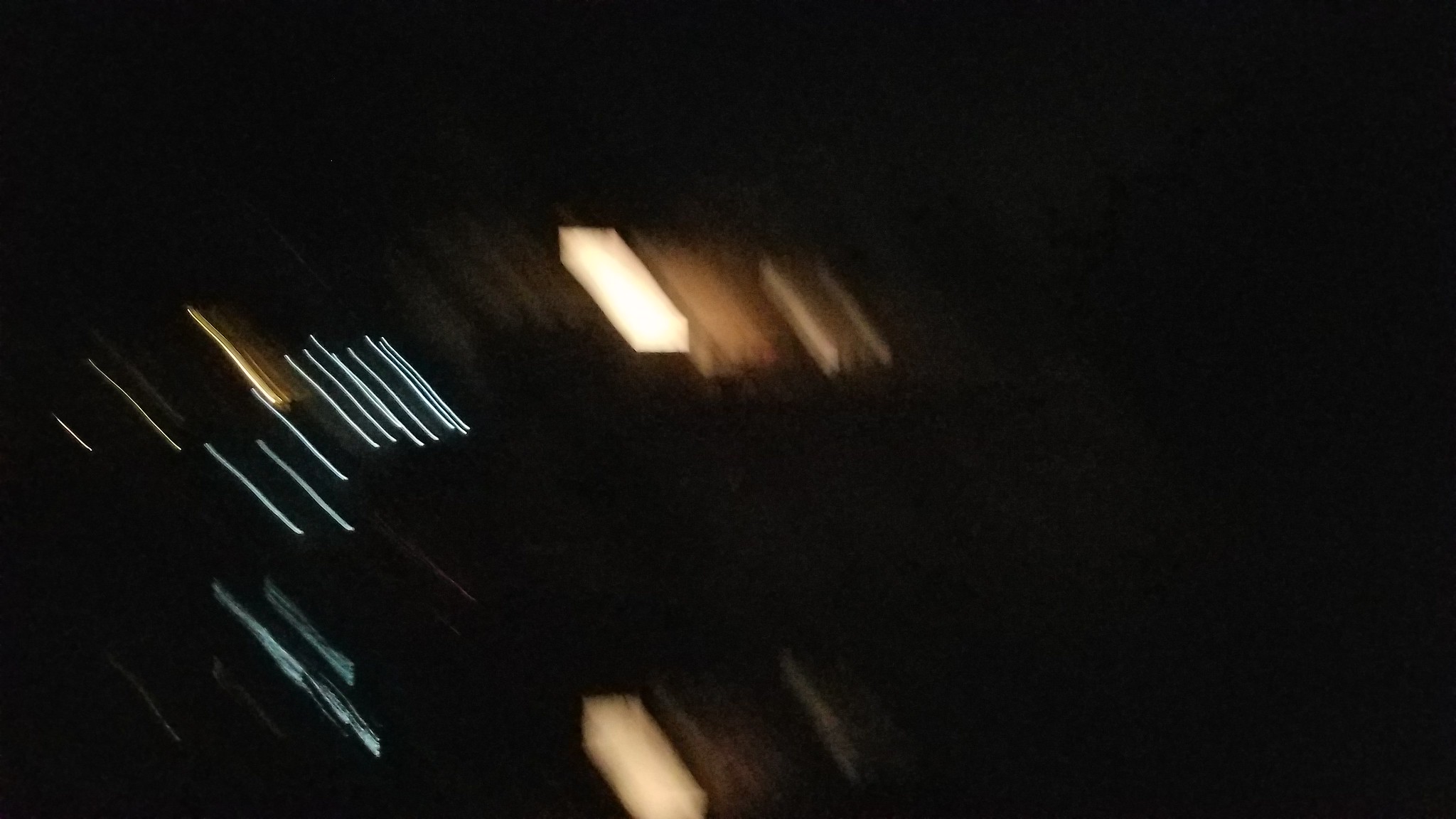The image is a very dark, blurred photograph captured with significant camera movement, leading to a predominant blackness on the top and right sides. The left side features wispy and blurry streaks of white and blue lights, resembling shooting stars. Towards the center bottom, a large tan rectangular light appears alongside an outline of what looks like a window, accompanied by darker gray structures that resemble shutters. In the middle and top center, there are additional tan rectangular lights adjacent to light brown window-like outlines and dark gray, shutter-like rectangles with white lines bordering the left and right. The overall lighting pattern appears to be diagonal, slanting from the upper left to the lower right, adding to the impression of motion and dynamic light trails in the scene.